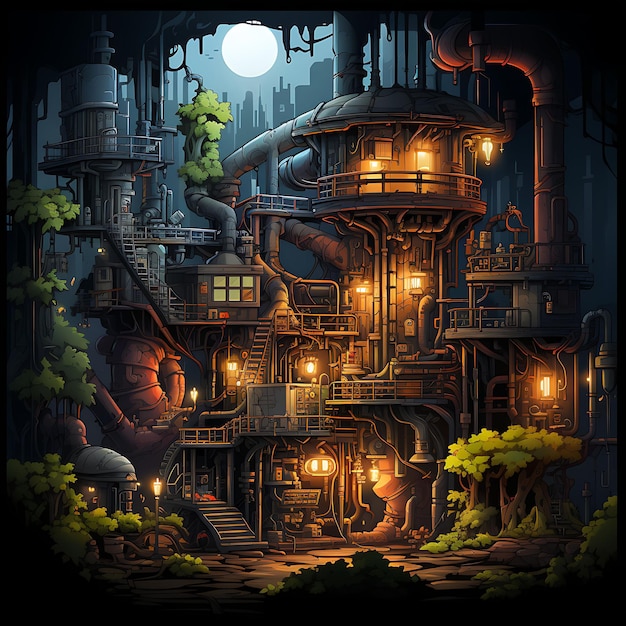The detailed, animated image resembles a steampunk-inspired treehouse or multi-level structure with a distinctive blend of futuristic and historical elements. The scene, predominantly black around the edges, features a night-time setting illuminated by a white, round moon positioned in the upper left. The structure, seemingly a mix of a treehouse and factory, consists of four to five stories connected by a series of winding stairs and platforms. The lower left corner shows the base stairs which lead to successive levels, each adorned with lanterns emitting a warm, yellow light. Additional cylindrical towers are visible on the upper portions, with interconnected pipes and vents, some of which are overgrown with vines. The bottom part of the image is entrenched with green leaf trees and a stone walkway, while more trees are scattered on the lower right side. There is a cityscape silhouette in the background under a bluish sky, and a few birds are in flight. The structure is dotted with lights including torches at the base and lamps throughout the platforms, creating a whimsical glow. A small shed-like extension is present on the left side of the main house, which is surrounded by vinery and additional signage near the stairway.